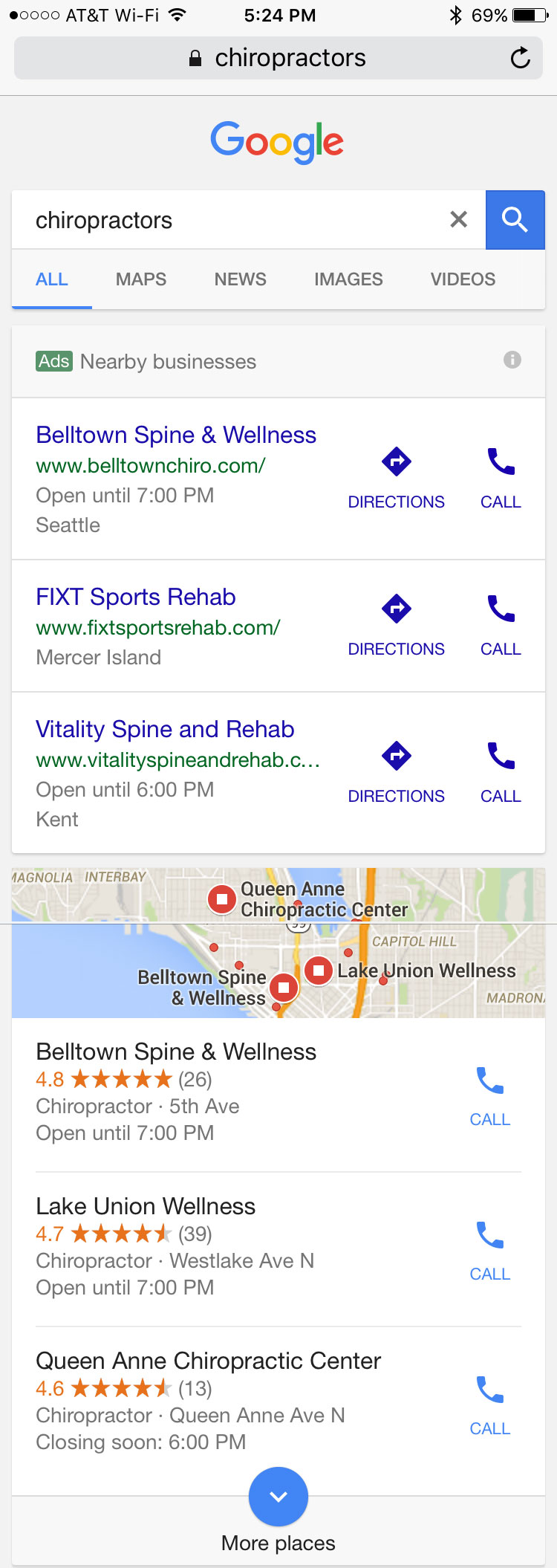This is a screenshot of Google search results for "chiropractor". The search displays several chiropractic services located near the user. The first result is Belltown Spine and Wellness in Seattle, which is open until 7 PM. Another nearby option is Fixed Sports Rehab on Mercer Island, though its hours of operation are not listed. Vitality Spine in Kent appears in the search results and is open until 6 PM. Additionally, Lake Union Wellness and Queen Anne Chiropractor Centre on Queen Anne Avenue North, which closes at 6 PM, are also shown. Each listing includes a phone number and a few have directions available.